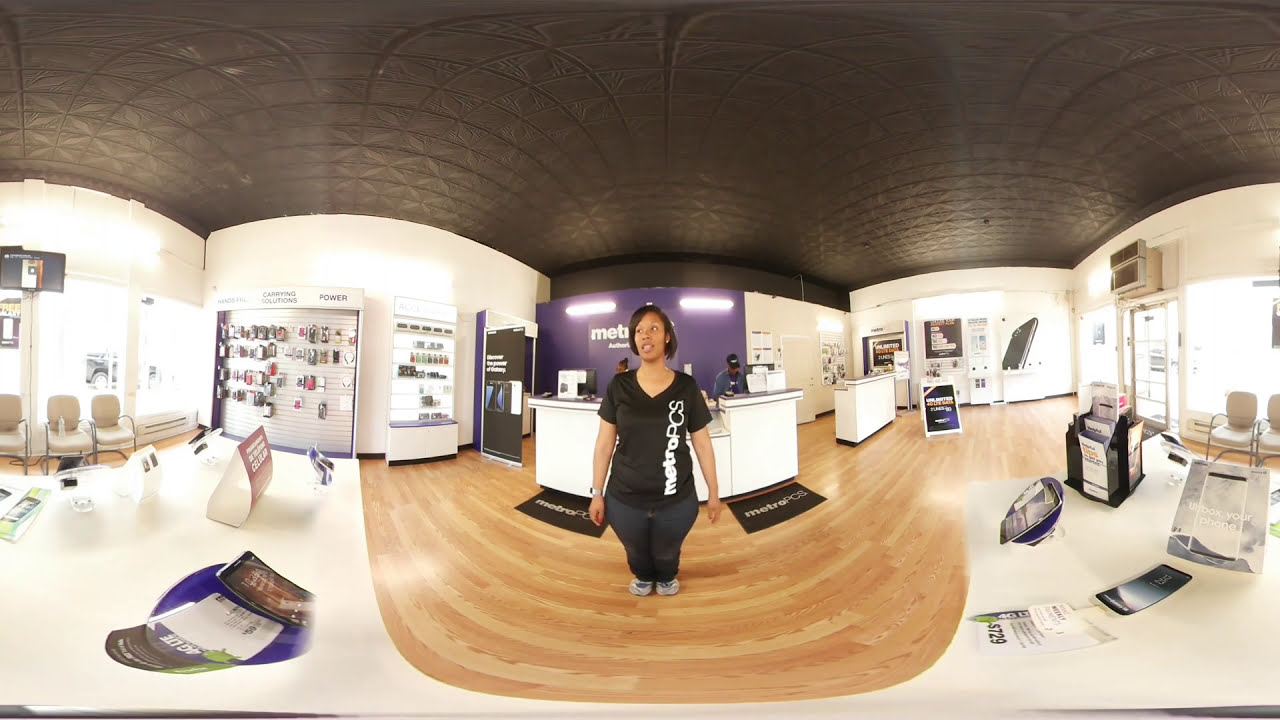In this 360-degree view of a Metro PCS store, a woman stands at the center wearing a black t-shirt with "Metro PCS" in white lettering running up the right side, paired with black pants and white sneakers. She has chin-length dark hair and her arms rest by her sides as she looks to the left. Behind her, two employees are visible at a large desk, one male and one female. The store features a blend of white and purple walls, adorned with various phone cases and promotional materials. The wooden floor, with its light brown and yellow textures, is complemented by two small black floor mats, each branded with "Metro PCS" in white letters. White chairs are available for customers along the left side of the room.